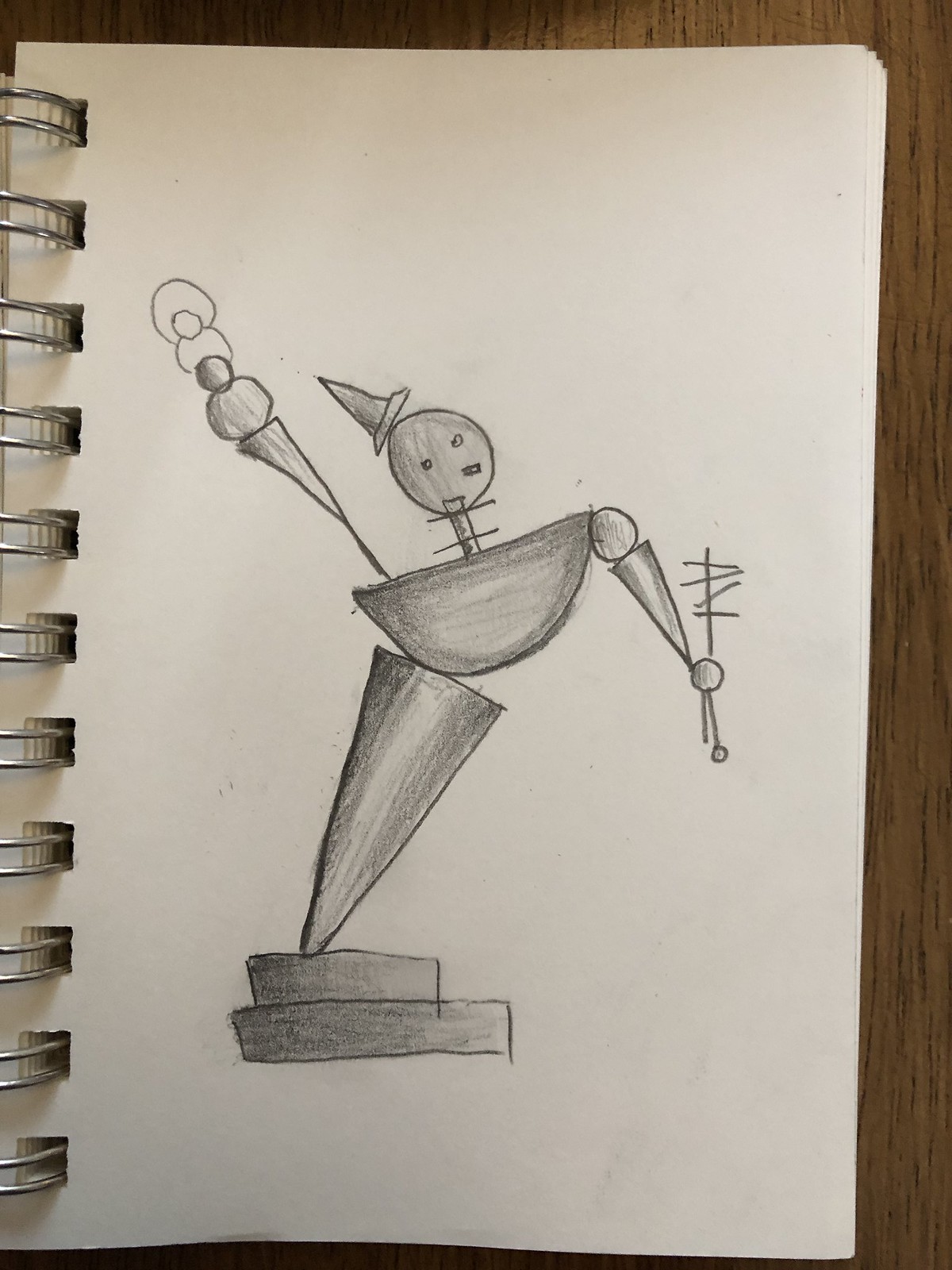This photograph features an unconventional, shape-based figure resembling a dancing puppet or robot. Designed entirely from geometric forms, the figure lacks typical humanoid proportions, lending it an eccentric appearance. The face is a simple circle adorned with a hat that strikingly resembles a traffic cone. A cylindrical neck supports the head, giving it a distinct, mechanical look. The body is depicted as a half-circle, adding to its abstract form. The right shoulder is marked by a circle, with the arm extending out as a pointed cone. In contrast, the left arm broadens outward like an ice cream cone, creating an asymmetrical design. The legs consist of large triangular cones, grounding the figure as it stands on a series of rectangular steps.